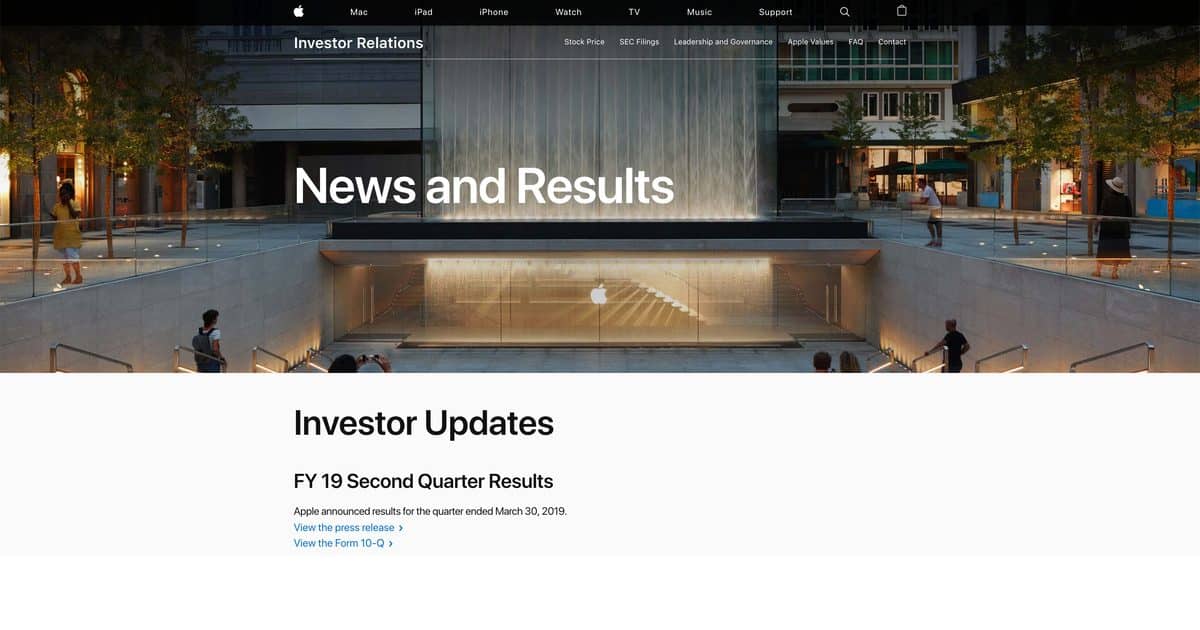Here is a cleaned-up and detailed caption based on the provided description:

---

Screenshot of the Apple Inc. investor relations homepage:

- **Top Border**: A half-inch black border spans the top section. Two-inch margins on both the left and right sides are empty.

- **Navigation Bar**: Starting from the left:
  - A white Apple logo.
  - White text with the following categories: "Mac," "iPad," "iPhone," "Watch," "TV," "Music," and "Support."
  - A search icon followed by a white-bordered square.

- **Main Image**: The central part of the page features a large image:
  - **Waterfall**: At the center of the image.
  - **Buildings**: Slightly visible on the left and right.
  - **Trees**: Flanking the image approximately two inches from both sides.
  - **People**: A person in a yellow shirt on the left, another person on the right, and several top portions of heads along the bottom.

- **Top Left Section**: Below the Apple emblem:
  - **Title**: "Investor Relations" in bold white text.
  - **Clickable Links**: Six clickable words in small white font.

- **Main Content**: Centered within the image:
  - **Headline**: "News and Results" in large, bold, white text.

- **Bottom Section**:
  - **White Border**: Approximately two inches from the left, a white border spans the section.
  - **Subheading**: "Investor Updates" in bold black text.
  - **Quarter Results**: Below the subheading, "FY19 Second Quarter Results" in smaller, but still bold, black text.
  - **Announcement**: "Apple announced results for the quarter ended March 30, 2019" in small black font.
  - **Links**: Two clickable blue links: "View the press release" and "View the Form 10-Q."

---

This cleaned-up caption ensures clarity and provides a thorough description of the webpage's layout and content.